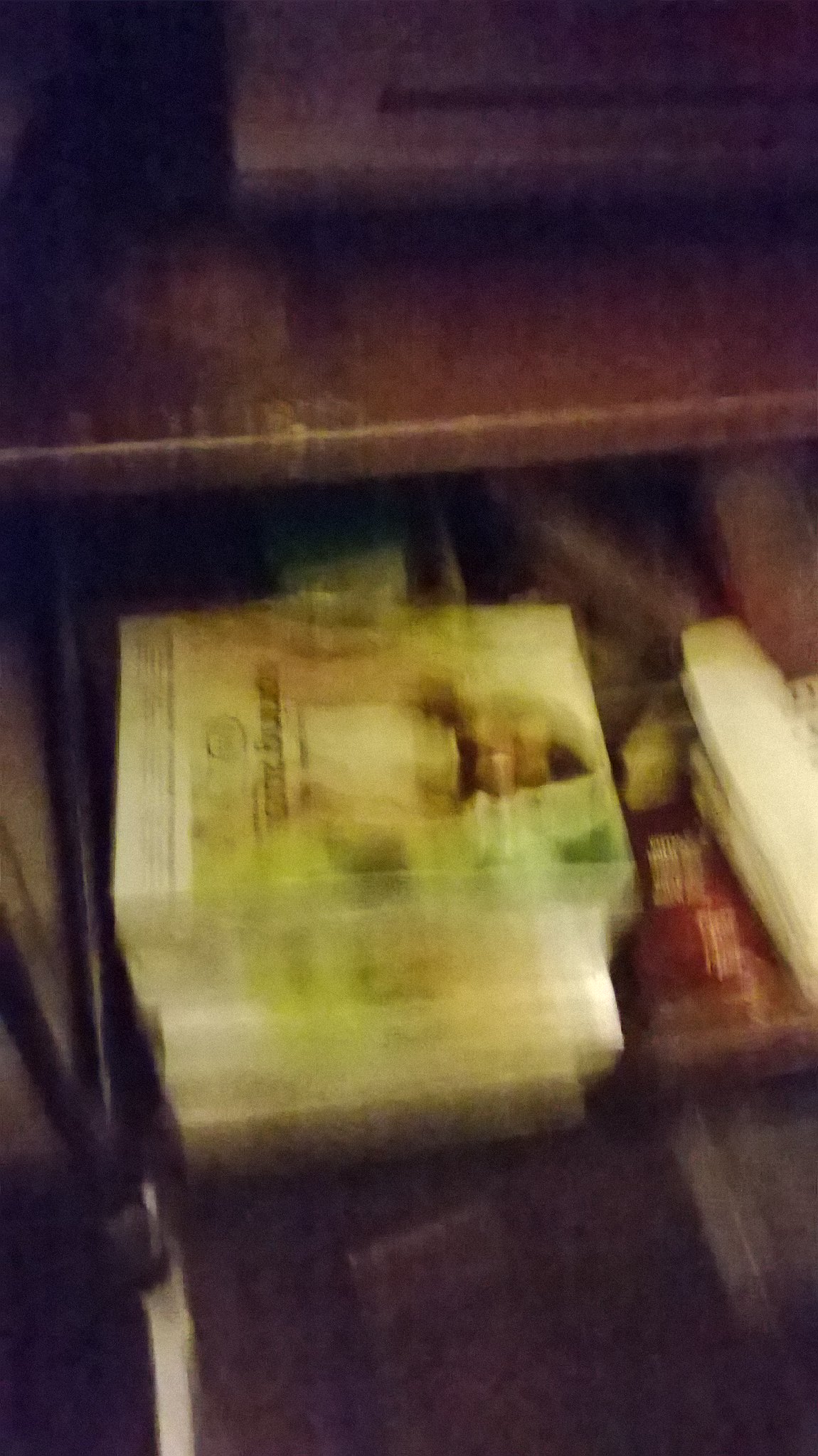In this blurred image, a dark wood stand with multiple shelves occupies the frame. At the top of this wooden cabinet sits a machine or device, although its details are obscured. The bottom shelf is stacked with what appear to be heavy items, possibly books or stacks of white papers. The topmost item in the stack features a cover with an image and some text, though it remains indistinct due to the blurriness. The floor area is partially visible, revealing the stand's black support bars and small wheels, indicating the stand's mobility.